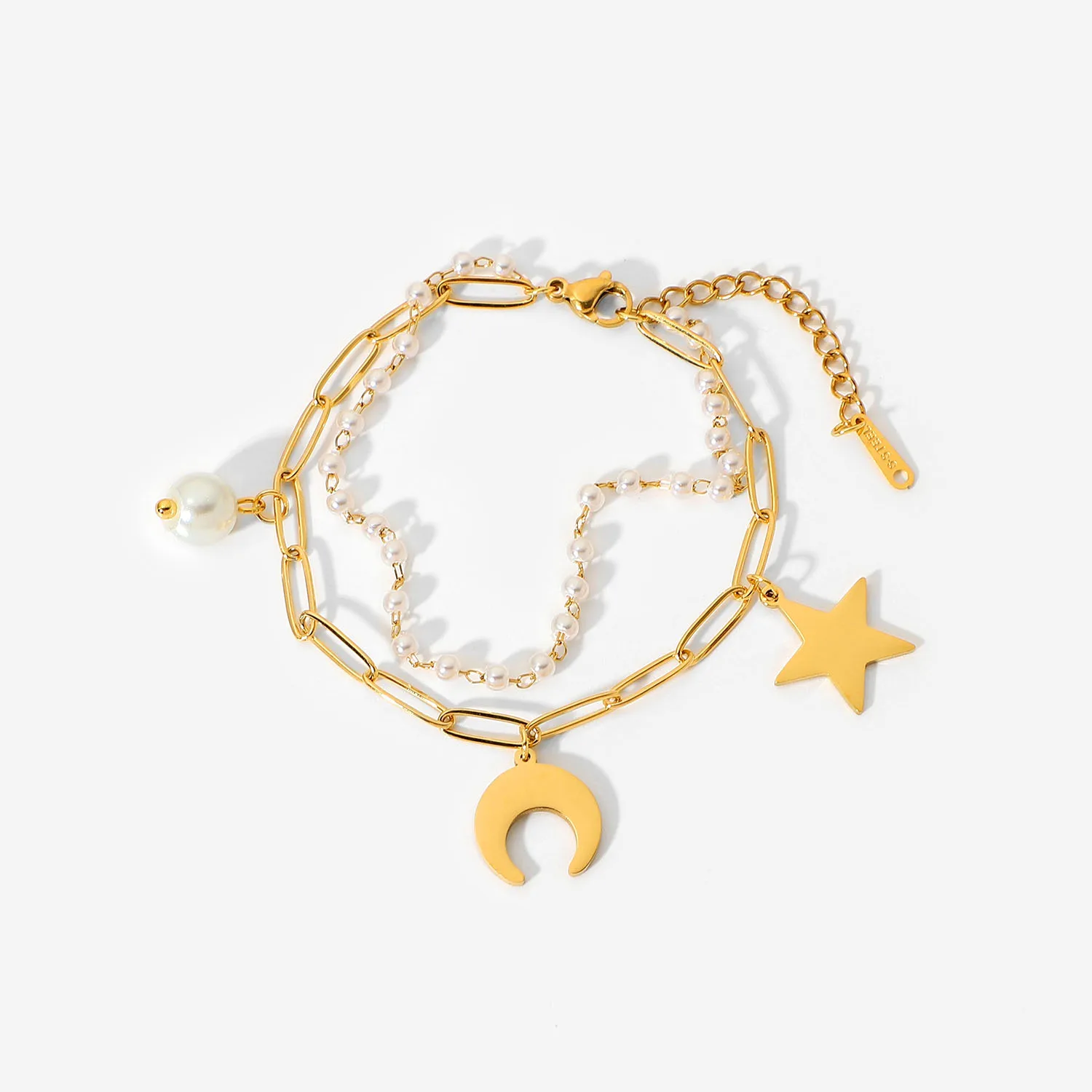In this detailed depiction of the jewelry piece, we have a gold-colored charm bracelet or necklace, meticulously adorned and centered against a blank, white background. The main segment of this piece comprises larger oval-shaped links, interspersed with a secondary chain made of smaller oval-shaped links featuring small, partly transparent round objects. Among the notable charms attached are a golden star-shaped symbol, a golden crescent moon symbol, and varying sizes of pearl-like elements, with one larger pearl adorning the main chain. The design is further enhanced by additional decorative components resembling paperclips, adding a unique touch to the overall aesthetic. The coloration of the piece includes shades of gold and white, with a hint of gray from shadows. The jewelry is finished with a small clip or hook at the top, ensuring it can be fastened securely.